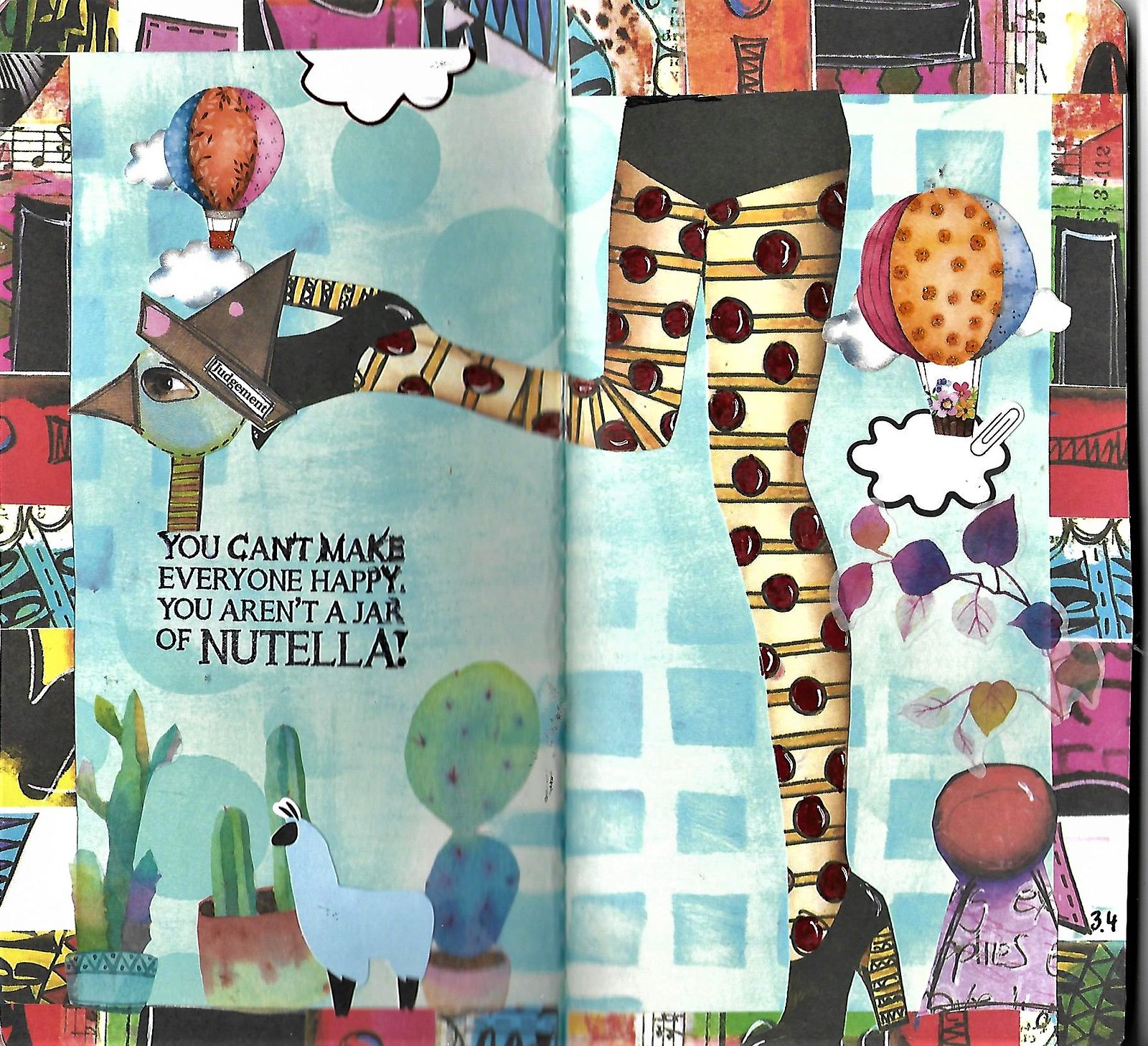The image is a vibrant, mixed-media art illustration designed like a page from a scrapbook or magazine, with a visible spine down the center. Set against a blue background, it prominently features a drawing of a woman's lower body adorned in black shorts and black high-heeled shoes. She is wearing alternating brown and white, and brown, white, and black leggings detailed with gold horizontal lines and a cherry pattern running from her upper thighs to her ankles.

To the left of her, an ostrich with a blue face and a triangular party hat is depicted with a brown beak and a single large eye. Above the ostrich's head is a flight balloon, and below it is the quote: "You can't make everyone happy; you aren't a jar of Nutella." 

The composition includes several other whimsical elements: a cactus growing from the bottom left, a bluish-grey llama in front of the cactus, and on the right, another hot air balloon in blue, orange, and pink carrying a bouquet of flowers. Additionally, a red apple is placed on a small platform at the bottom right corner, surrounded by indeterminate red, green, and black objects scattered across the image. Musical notes appear on the left-hand side, and random color splotches and line drawings fill the border, creating an eclectic, colorful collage effect. 

This extravagant interplay of characters, quotes, and patterns makes the image a visually intriguing promotion, potentially linked to the Nutella brand.